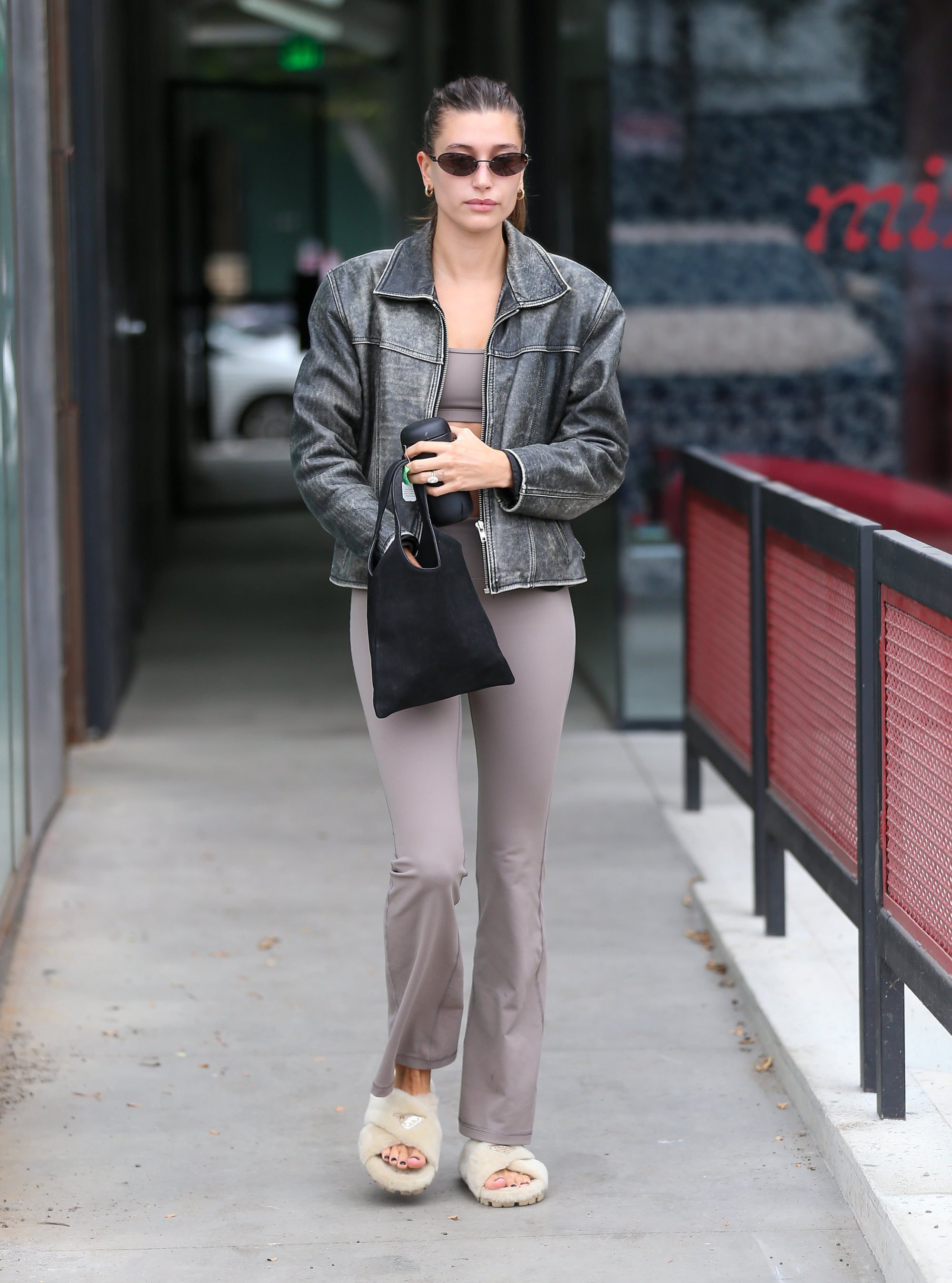In this image, a stylish woman is walking along a concrete walkway that appears to be an outside hallway between two sections of a building. The woman, possibly in her late 20s to early 30s, exudes a sense of celebrity or artistic flair. She is a white woman with black hair pulled back into a ponytail, and she is dressed in a black distressed leather bomber jacket reminiscent of World War II pilots. Under the jacket, she wears a purple-beige tank top, and she pairs it with light gray, comfortable yet business-like pants that resemble pajama pants in their softness. She has white slipper-type shoes that intriguingly blend casual comfort with a hint of business style. Dark oval sunglasses shield her eyes. 

In her left hand, she holds a smartphone and has a ring on her wedding finger. Her right hand is immersed in a small black purse, as if searching for something. To her right, a black frame fence with red grating provides a vivid contrast to her ensemble. The walkway leads to a blurred white car in the background, and towards the upper right, a tan vehicle and red letters "M-I" are visible. The overall color theme of the scene includes shades of red, white, gray, and black, punctuated by the woman's chic attire. No other people are present in the frame.